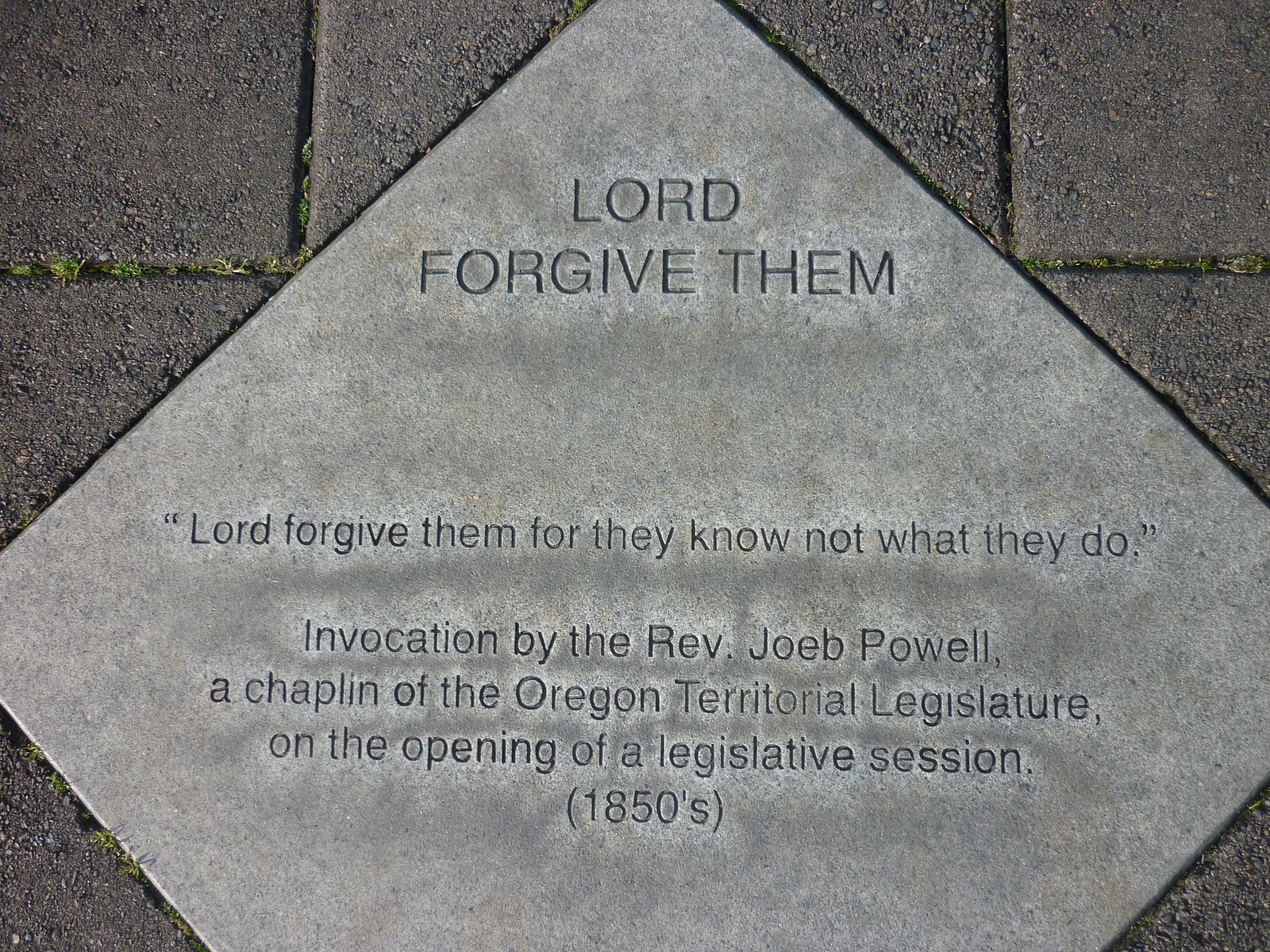The image is a landscape-oriented color photograph showcasing a memorial plaque installed within a walkway of bricks. The plaque is a gold-colored concrete square, positioned diagonally to appear diamond-shaped, partially cropped at both the top and bottom edges. It is set amidst darker concrete bricks, some of which have grass growing between their cracks, indicating its placement on the ground. The engraving at the top of the plaque, in all caps, reads, "LORD FORGIVE THEM." Beneath this, in the center of the plaque, is the quote, "LORD FORGIVE THEM, FOR THEY KNOW NOT WHAT THEY DO." Following the quote is an attribution: "INVOCATION BY THE REVEREND JOAB POWELL, A CHAPLAIN OF THE OREGON TERRITORIAL LEGISLATURE, ON THE OPENING OF A LEGISLATIVE SESSION, 1850S." This detailed commemoration integrates historical and biblical references, creating a solemn and thoughtful presentation.